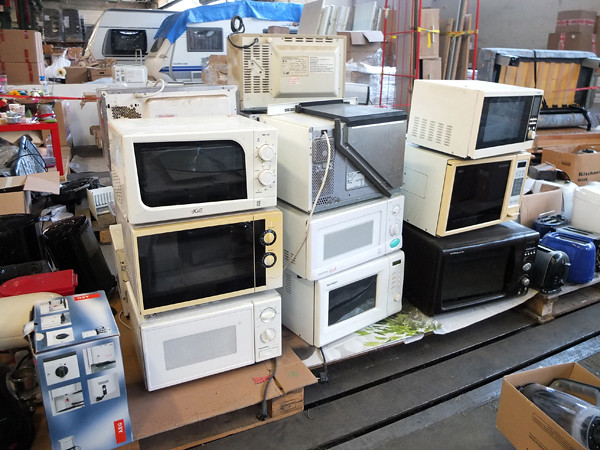The photograph captures a cluttered indoor space that appears to be a storeroom, repair shop, or junk room, filled primarily with stacks of microwave ovens. Centered within the image are three distinct stacks of microwaves, each stack comprising three units. The left stack features a white microwave on the bottom, a yellow one in the middle, and a white microwave on top. Moving to the middle stack, the configuration includes a white microwave at the bottom, another white microwave with turquoise knobs in the middle, and the back of a gray microwave with a white side on the top. To the right, another stack shows a black microwave at the bottom, a yellow and white microwave in the middle, and a white microwave on top.

The microwaves, likely from the mid to late 1980s, exhibit various states of wear and different colors, like white, yellow, and black. The lower right of the scene includes a cardboard box, while a red, white, and blue box sits adjacent to the left stack of microwaves. Scattered around the space are various unidentifiable pieces of equipment and miscellaneous items, contributing to the disorganized appearance. Notably, in the background, a set of red, thin items resembling a ladder is visible, and further to the left, the side of a camper can be seen. A piece of furniture is also visible in the upper right corner, turned upside down to reveal its underside. The entire scene is set on a dark wooden floor, with gaps visible between the slats.